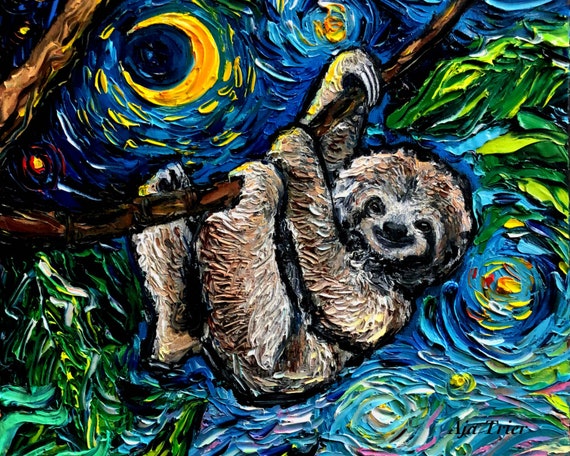This painting features a sloth hanging from a medium-sized brown branch, set against a background reminiscent of Van Gogh's "Starry Night." The sloth, positioned centrally, appears to be smiling, with distinctive black markings around its mouth, nose, and eyes, as well as white fur surrounding its face. The forehead displays a mix of black, light brown, and white hues. The sloth's arms and legs, which grasp the branch, are painted in shades of brown and white, and its hands are accentuated by large white claws. The night sky background is rich with swirled strokes of dark blue paint, integrating a yellow crescent moon in the upper left corner. Additional elements include green leaves in the bottom left and an artist's watermark, "Aja Trier," in black text at the bottom right.